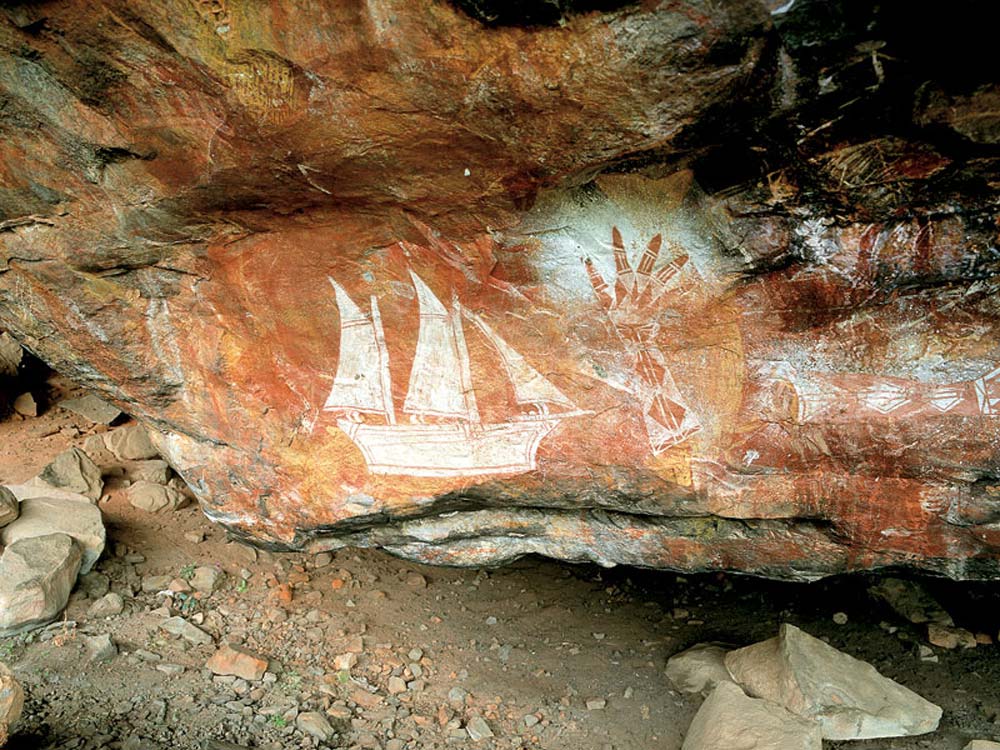The photograph captures a highly detailed section of a grayish-greenish-brown cave wall adorned with intriguing petroglyphs. Dominating the scene is an impressive white drawing of a three-masted wooden ship, positioned on the left side of the stone. The ship’s striking sails and intricate design suggest a significant level of craftsmanship. Adjacent to the ship, on the right, is a meticulously depicted human hand up to the elbow, richly adorned with diamond-shaped patterns and linear designs in both brown and white, which gives the appearance of possible tattoos or ornamentations. The reddish-brown hues on the side of the stone add further depth and contrast to the imagery. Though the origins of these petroglyphs are uncertain, whether ancient or contemporary, the detailed and vivid nature of the artwork renders the cave wall an extraordinary example of human expression and art.